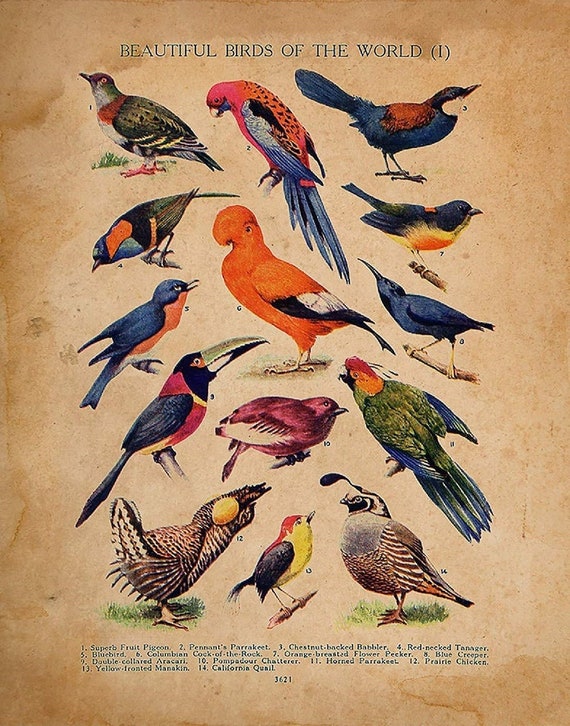This vertical educational poster, titled "Beautiful Birds of the World I," features meticulously illustrated birds on a beige, antiqued background, hinting at its age with visible stains and watermarks. The vivid illustrations, possibly drawn with colored pencils or painted, display 14 different bird species, each facing various directions and showcasing vibrant colors. Notable birds include the Superb Fruit Pigeon with green, orange, brown, and white plumage; the pink and orange Penance Parakeet with black, white, and purple wings; an orange bird with black and white feathers situated centrally; a red, black, and white-beaked Toucan; an all-black Crow with yellow feet; and a yellow, black, and red bird resembling a sparrow. Accompanying the illustrations, a numbered list at the bottom provides the names of each bird: 1. Superb Fruit Pigeon, 2. Penance Parakeet, 3. Chestnut-backed Babbler, 4. Red-necked Tanager, 5. Bluebird, 6. Colombian Cock-of-the-rock, 7. Orange-breasted Flowerpecker, 8. Blue Creeper, 9. Double-collared Aracari, 10. Pompadour Cotinga, 11. Horned Parakeet, 12. Prairie Chicken, 13. Yellow-fronted Manakin, and 14. California Quail. This poster appears to be from an ancient, comprehensive encyclopedia, as indicated by the page number 3621.